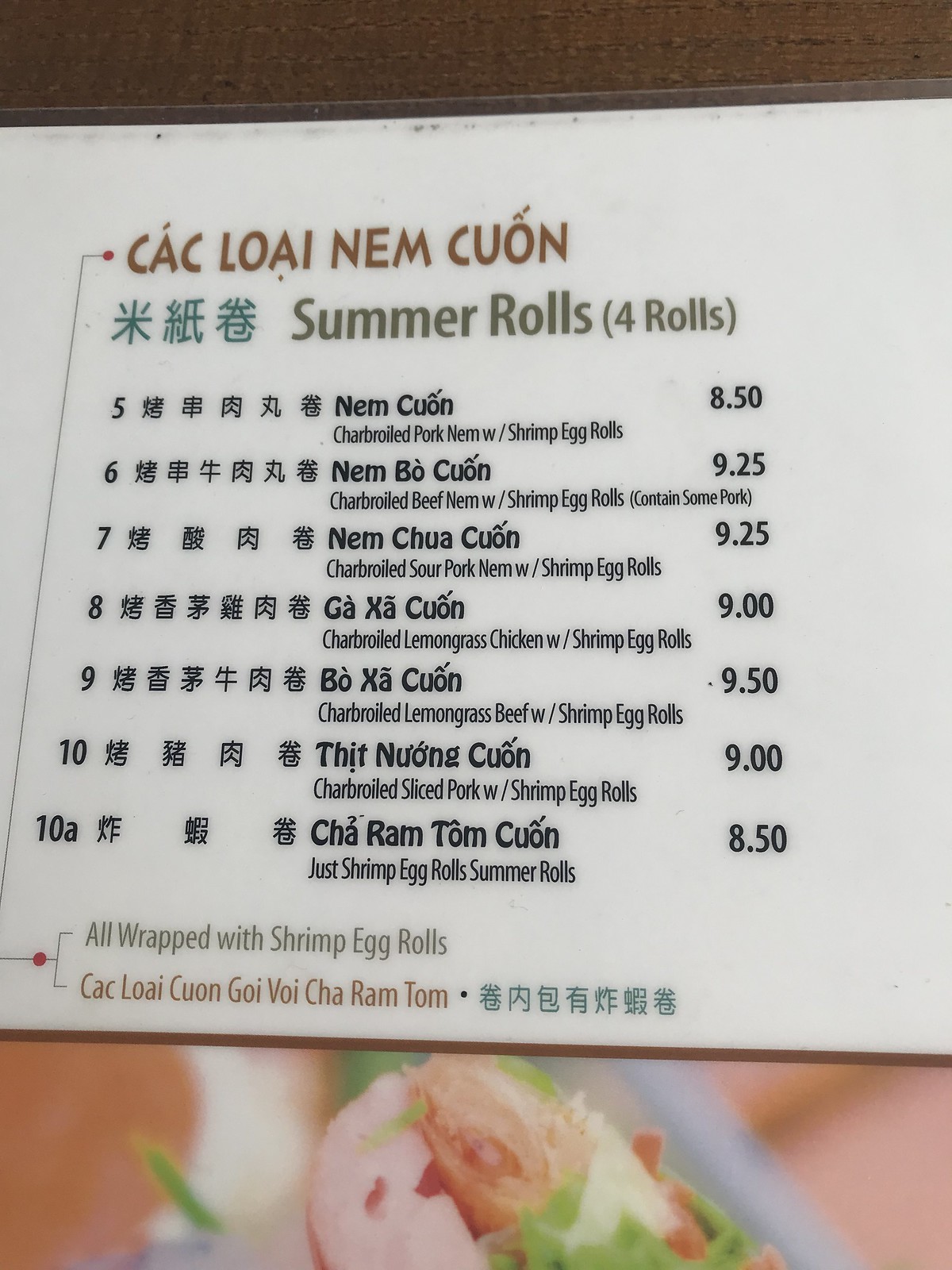This detailed image is of a laminated menu, specifically focusing on the summer rolls section. The top two-thirds of the menu features a white background with textual content. Beneath this section, a summer roll is partially visible, angled slightly to the right near the center of the frame. 

The background to the left of the summer roll transitions from a pinkish hue to a lighter pink towards the right. A single green leaf can be seen in the middle of this gradient. Towards the right side of the summer roll, there's a noticeable gray piece that stretches diagonally from the top left to the bottom right, surrounded by more pink.

The exterior of the summer roll is pink, while the interior displays a variety of colors including light pink, green, and yellow. Just above the summer roll, the brown laminate reveals a hint of a table beneath. In reddish-brown letters, the text "C-A-C-L-O-A-I-N-E-M-C-U-O-N" is visible, followed by three Chinese characters underneath. To the right of this, in black text, it reads "Summer Rolls," with a note indicating that there are four rolls. 

Under this heading, the menu is numbered from 5 to 10, continuing with 10A. The dish names are listed to the right of these numbers, and the prices are further to the right. A note at the bottom mentions that all rolls are wrapped with shrimp egg rolls, with this information repeated in a foreign language. 

The summer roll image begins beneath this text, showcasing the details described above.